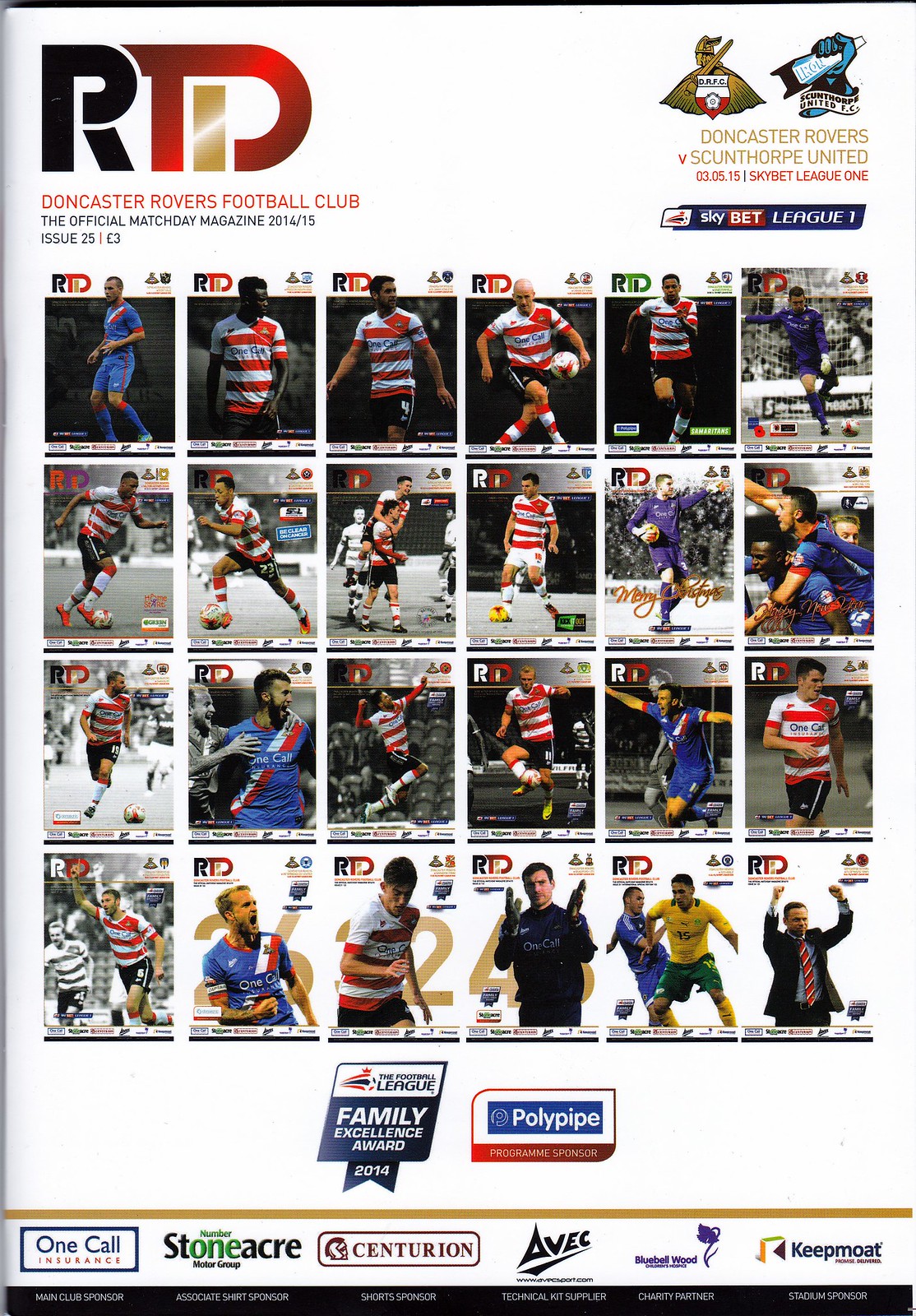The image is the colorful cover of the Doncaster Rovers Football Club's official Match Day magazine, issue 25, from the 2014/15 season, priced at three pounds. The top features a prominent RTID logo in black and red, with "Doncaster Rovers Football Club" just below it. The headlines proudly announce the match between Doncaster Rovers and Scunthorpe United, set for May 3, 2015, in the SkyBet League One. The center of the magazine displays five rows of six squares, each showcasing detailed photos of players in action, wearing uniforms of white shirts with red stripes or blue shirts with a diagonal white and red stripe. Sponsor logos such as One Call Insurance, Stoneacre, Centurion, AVEC, Polypipe, and Keepmoat, as well as accolades like the Football League Family Excellence Award 2014, are displayed at the bottom, making the cover easy to read and richly detailed.